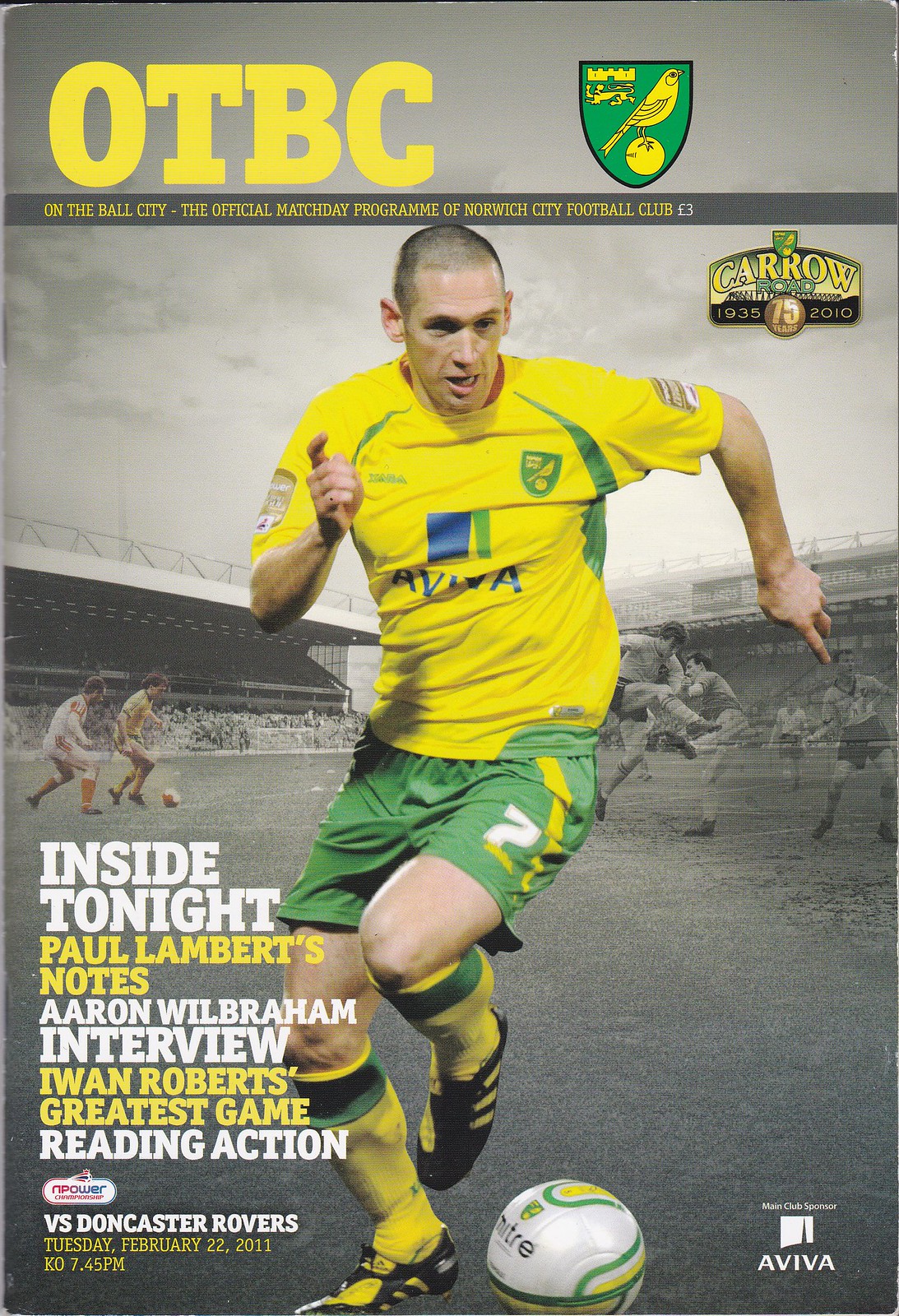The image depicts the vertically aligned rectangular cover of a soccer magazine, set against a gray background with grayish-white clouds at the top. Prominently featured in the upper left-hand corner in large, yellow, all-caps block letters is "OTBC," with a thin dark gray strip underneath displaying "On the Ball City, the official match day program of Norwich City Football Club" in yellow letters. Dominating the cover is a dynamic action shot of a man around 30 years old, wearing a yellow jersey, green shorts, and yellow and green socks. He is poised to kick a soccer ball with his left foot. Notable text on the left side near his knee includes "Inside Tonight" in white, followed by other highlights in alternating yellow and white text: "Paul Lambert's notes," "Aaron Wilbraham interview," "Iwan Roberts' greatest game," and "Reading action." At the bottom of the image, it reads "versus Doncaster Rovers, Tuesday, February 22, 2011" indicating the match date, and "KO 7:45 PM" for the kickoff time. Additionally, in the lower right-hand corner, there is a logo with the name "Aviva" in white letters.